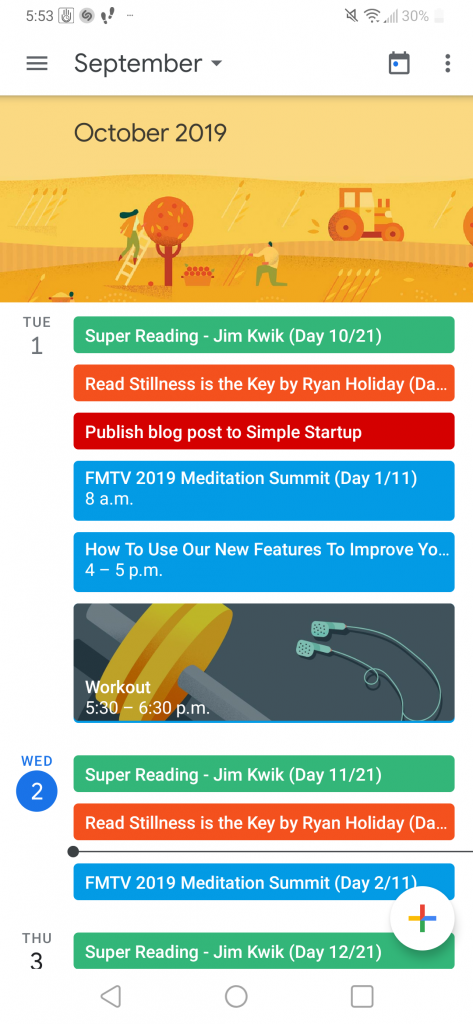This image, captured on a cell phone, shows a detailed digital calendar interface. The phone's status bar indicates a 30% battery life, a strong network connection, and that the sound is muted. The time displayed is 5:53, and the date is sometime in September. The interface includes a box with three vertically aligned dots and a separate icon featuring three horizontal lines on the left side.

A photograph within the calendar, labeled "October 2019," showcases a serene farm scene where people are busy picking apples. A tractor is visible in the background, and fields stretch out under a clear sky. Among the workers, a man is kneeling, possibly gathering apples or tending to crops.

The calendar entries reveal a structured schedule filled with various activities. On Tuesday, October 1st, noteworthy entries include:

- **Super Reading with Jim Quick:** Day 10 out of 21
- **Reading Assignment:** "Stillness is the Key" by Ryan Holiday
- **Blog Posting:** Publish a post to Simple Startup
- **FM TV Meditation Summit 2019:** Day 1 of 11, at 8 a.m.
- **New Features Training:** 4 to 5 p.m.
- **Workout Session:** 5:30 to 6:30 p.m.

Wednesday, October 2nd, continues the structured routine with:

- **Super Reading with Jim Quick:** Day 11 out of 21
- **Reading Assignment:** "Stillness is the Key" by Ryan Holiday
- **FM TV Meditation Summit 2019:** Day 2 of 11

Thursday, October 3rd, lists:

- **Super Reading with Jim Quick:** Day 12 out of 21

The calendar employs a color-coding system, using shades of green, red, and blue to differentiate between various types of activities and tasks. This meticulous and colorful layout exemplifies a well-organized agenda.